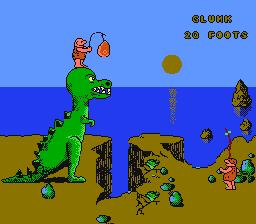In this vibrant video game scene, the background is dominated by various shades of blue, encompassing a serene blue sky that meets a calm blue lake. Gold letters at the top of the screen spell out "Glump, 20 ft." Below, a radiant yellow sun is depicted in the midst of setting, casting a warm hue over the tranquil water and the large gray rocks that jut out prominently. In the foreground, a small, angry-looking green dinosaur is being used as a perch by a small caveman. The caveman is holding a fishing pole with a red object dangling from the end. On the ground nearby, another small caveman stands watching the scene unfold. The brown terrain around them is scattered with green rocks and various small objects, adding texture and detail to the setting.